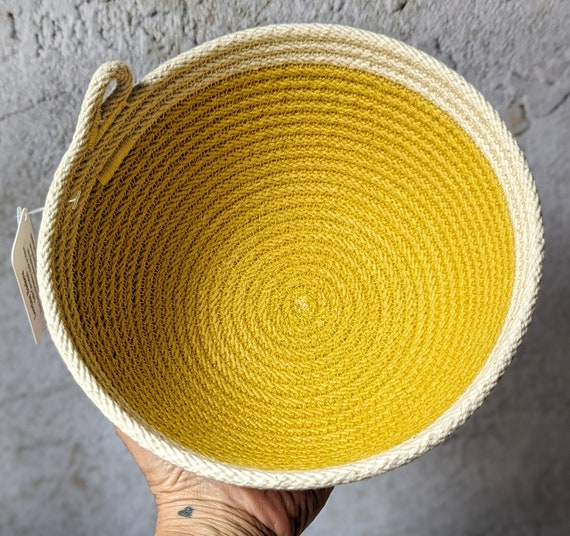This detailed image shows a hand holding a large, handcrafted woven bowl, most likely intended for sale as indicated by a visible tag on its side. The bowl is a striking combination of bright gold in the center, transitioning to off-white beige threading or rope along the outer rim. The person holding the bowl is identifiable by a small heart tattoo on the inside of their wrist. The background features a rough, grayish wall, suggesting a rustic or industrial setting, which complements the handcrafted aesthetic of the bowl. The perspective of the photo is angled downwards, emphasizing the craftsmanship and texture of the woven material.